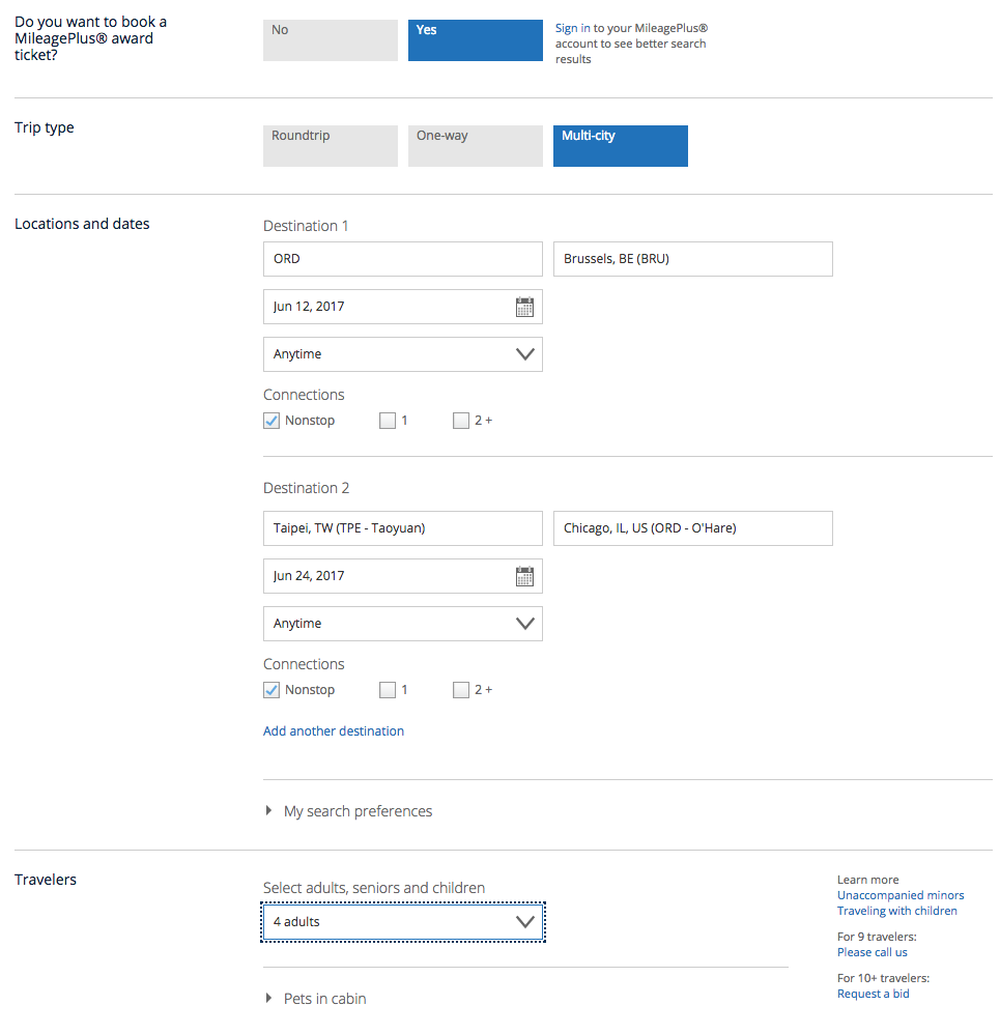A screenshot with a white background showcases a booking interface for a MileagePlus award ticket. It prominently features a question at the top: "Do you want to book a MileagePlus award ticket?" Below this, there are two options: a gray button labeled "No" and a blue rectangle labeled "Yes." Additionally, there is a prompt to sign in to your MileagePlus account for better search results, with "Sign in" highlighted in blue.

The interface allows for multiple trip types: round trip, one-way, or multi-city. The "Locations and Dates" section is also visible, with fields for specifying destinations and travel dates. 

For Destination 1, the information provided includes:
- Airport code: ORD or DRD
- Destination: Brussels, Belgium (BRU)
- Departure date: June 12, 2017
- Time: Any time
- Connections: Three checkbox options — "Nonstop" (checked), "1 Stop," and "2+ Stops"

For Destination 2, the details are as follows:
- Destination: Taipei, Taiwan (TPE)
- Return to: Chicago, Illinois (ORD)
- Return date: June 24, 2017
- Time: Any time
- Connections options: Same as for Destination 1

The layout is designed to assist in planning a round trip or multi-city travel, emphasizing customizable search filters for flights including flexible connection options.